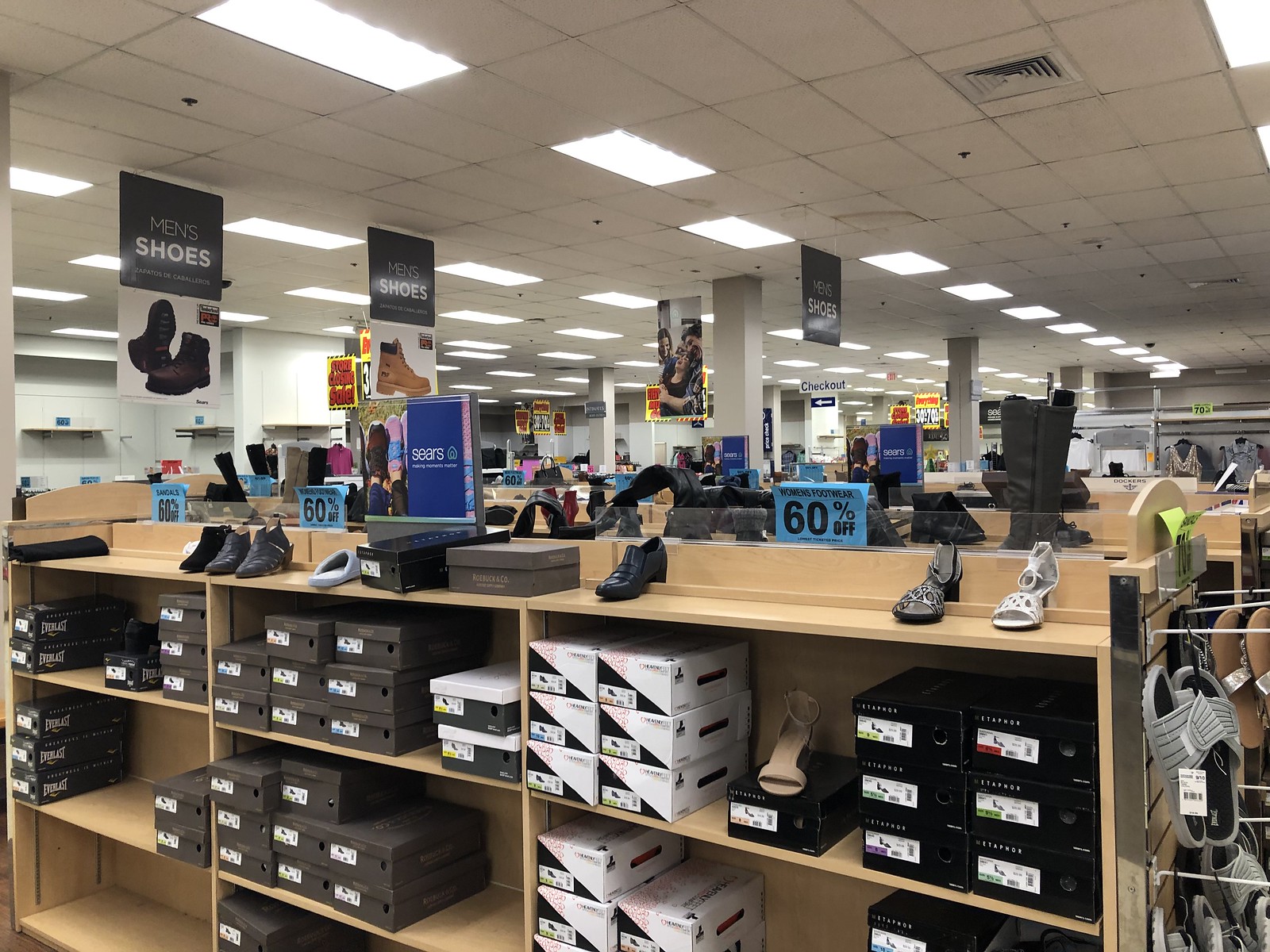This detailed interior photograph captures a shoe department within a Sears store. Prominently featured are light tan wooden shelves arranged diagonally across the scene, containing rows of shoe boxes in black, white, and brown. On the top shelf, various shoes are displayed with their toes pointing toward us, including open-toe sandals in white and leopard print, a tan woman's shoe, a slipper-style shoe, and black tennis shoes. The top shelf also sports a blue sign reading "60% off women's footwear." To the left, a large overhead sign designates the men's shoes section. The ceiling above showcases a grid-like pattern with fluorescent lights running horizontally and an air vent. Additional shoes, including small white Velcro slip-ons, hang from wire hooks attached to silver metal posts at the shelf's ends. The background reveals more shoes and some hanging clothing merchandise, emphasizing the store's extensive selection.